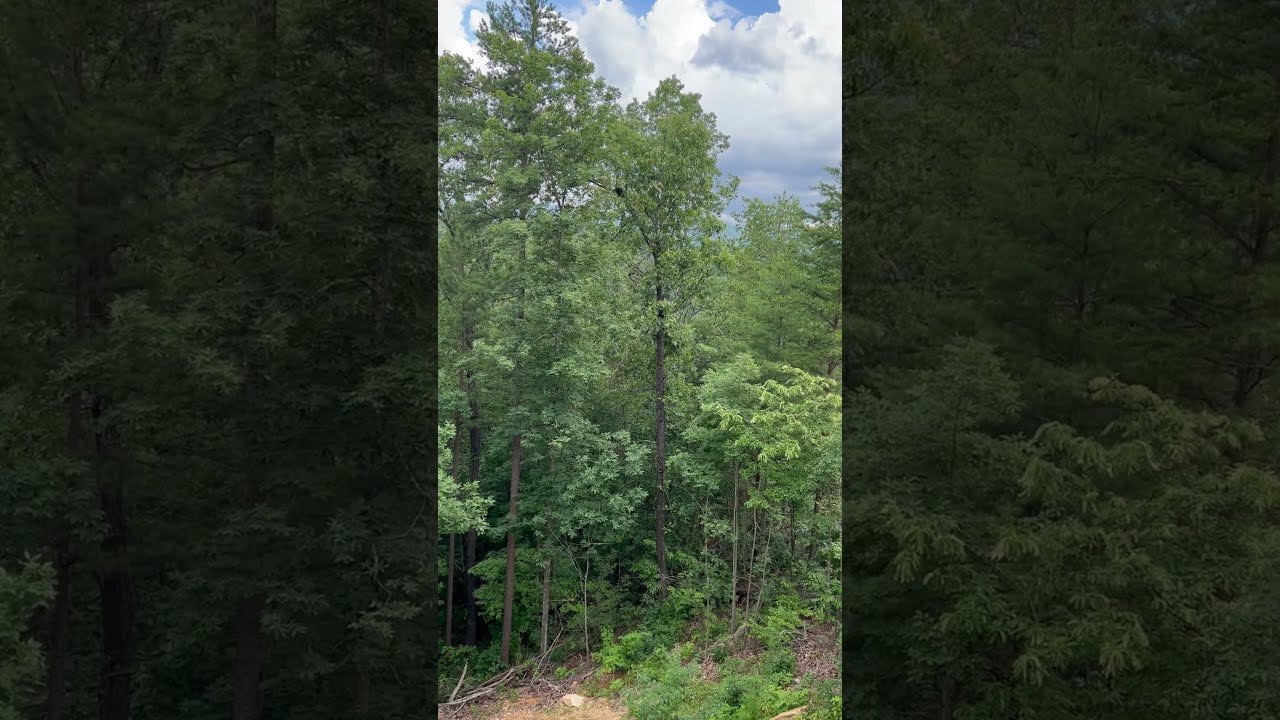This portrait-oriented photograph captures a serene and remote forest scene, dominated by a variety of deciduous trees that stretch from the ground to the top of the frame. These trees range in height and display a spectrum of leaf colors, from yellow-green to the deeper shades reminiscent of evergreen foliage. The forest floor, visible at the bottom of the image, is dotted with dirt, a rock in the lower left corner, and an array of fallen, leafless branches and decaying tree trunks. The sky above is a picturesque expanse of bright blue, interspersed with fluffy white clouds, some of which appear heavier and storm-like near the top right corner. The detailed scene is framed by wide borders on the left and right, consisting of magnified and grayed-out sections of the central image, creating a unique and artistic edge to the photograph. No humans or man-made objects are present, adding to the untouched and natural beauty of the setting.